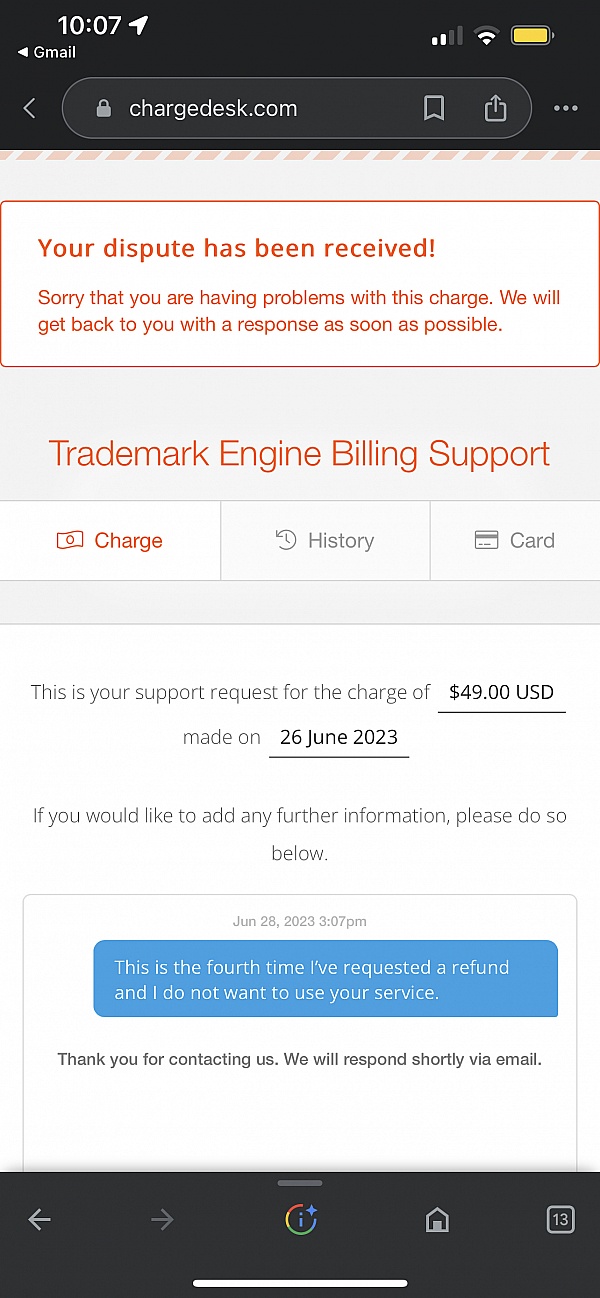The image displays a screenshot from a website with a black border at the top, featuring a URL bar showing "charredesk.com." Below the URL bar, there is a prominent rectangular white box outlined with a red border. Inside the box, a message reads: "Your dispute has been received. Sorry that you're having problems with this charge. We will get back to you with a response as soon as possible."

Beneath this message, in red text, it says "Trademark Engine Billing Support," followed by three buttons. The first button, labeled "Charge," is highlighted in red, while the other two buttons—"History" and "Card"—are in gray.

Further down, the text states: "This is your support request for the charge of 49 USD made on 26 June 2023. If you would like to add any further information, please do so below." Following this, there is a text or chat box displaying a blue bubble with the message: "This is the fourth time I've requested a refund and I do not want to use your service." 

Under this blue bubble, the text concludes with: "Thank you for contacting us. We will respond shortly via email."